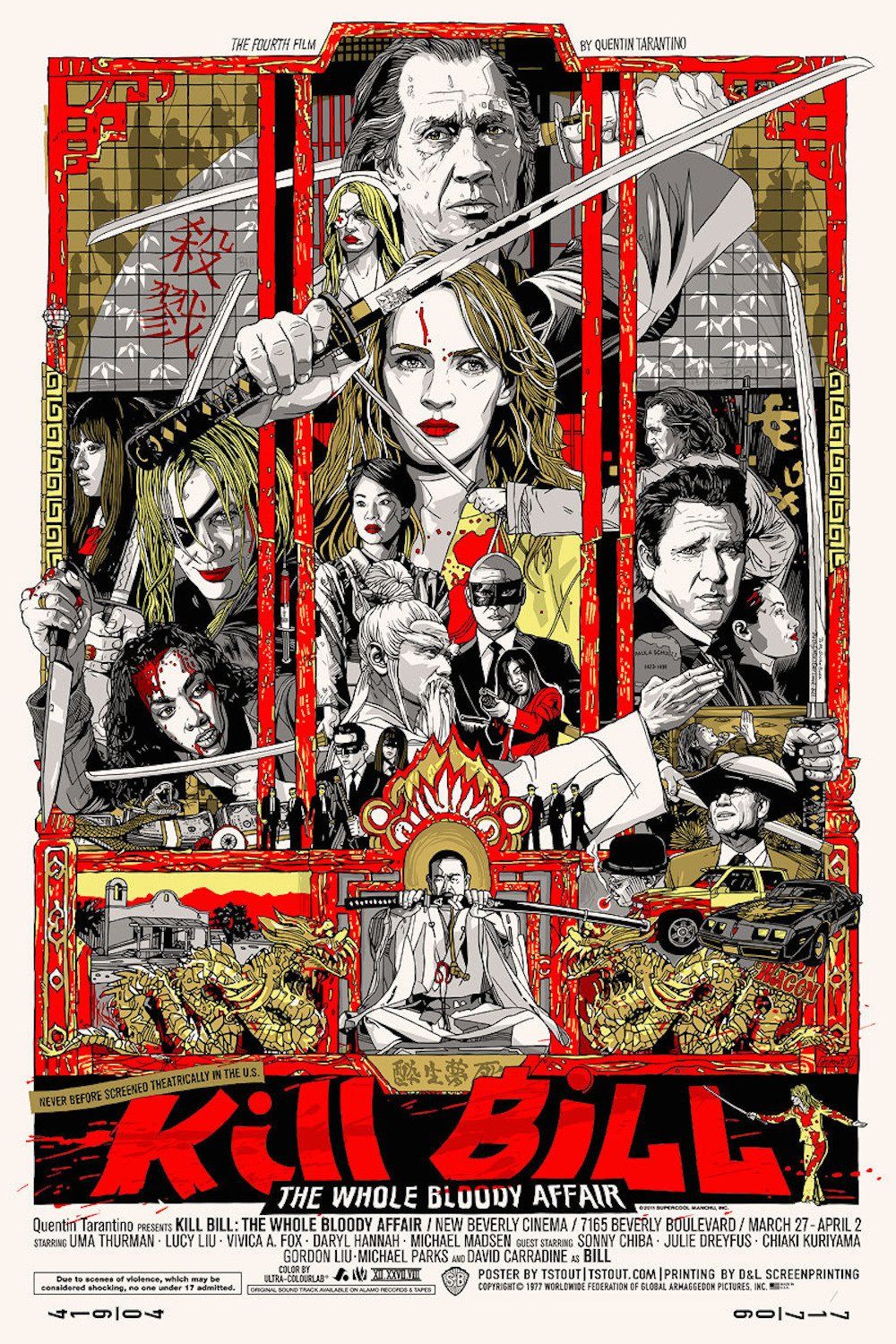This detailed movie poster for Quentin Tarantino's "Kill Bill: The Whole Bloody Affair" showcases an intricate blend of hand-drawn or digitally illustrated artwork. At the very top, in small black lettering, it announces "The Fourth Film by Quentin Tarantino." The central image is framed by a red and gold Asian-inspired border that mimics a Japanese rice paper wall. The poster features an elaborate, black-and-white collage of the film's characters, with notable splashes of color—such as Uma Thurman's red lips and the blood dripping from her forehead. She is depicted prominently wearing her iconic yellow suit, splattered with blood, and holding a samurai sword, poised for battle. 

The artwork also includes various characters armed with swords and weapons, alongside other thematic elements like dragons and scenes from the movie. At the bottom, large red letters spell out "Kill Bill," with "The Whole Bloody Affair" written below in white on a black background. Underneath this, the credits detail the showing at New Beverly Cinema from March 27th to April 2nd at 7165 Beverly Boulevard. 

The overall design suggests a high level of craftsmanship, with a rich color palette featuring reds, yellows, and browns, likely indicating that this is a specialized poster, possibly created by the company Mondo known for their elaborate movie posters. The collage of faces and scenes effectively captures the essence of the film's revenge-driven narrative and samurai influences.